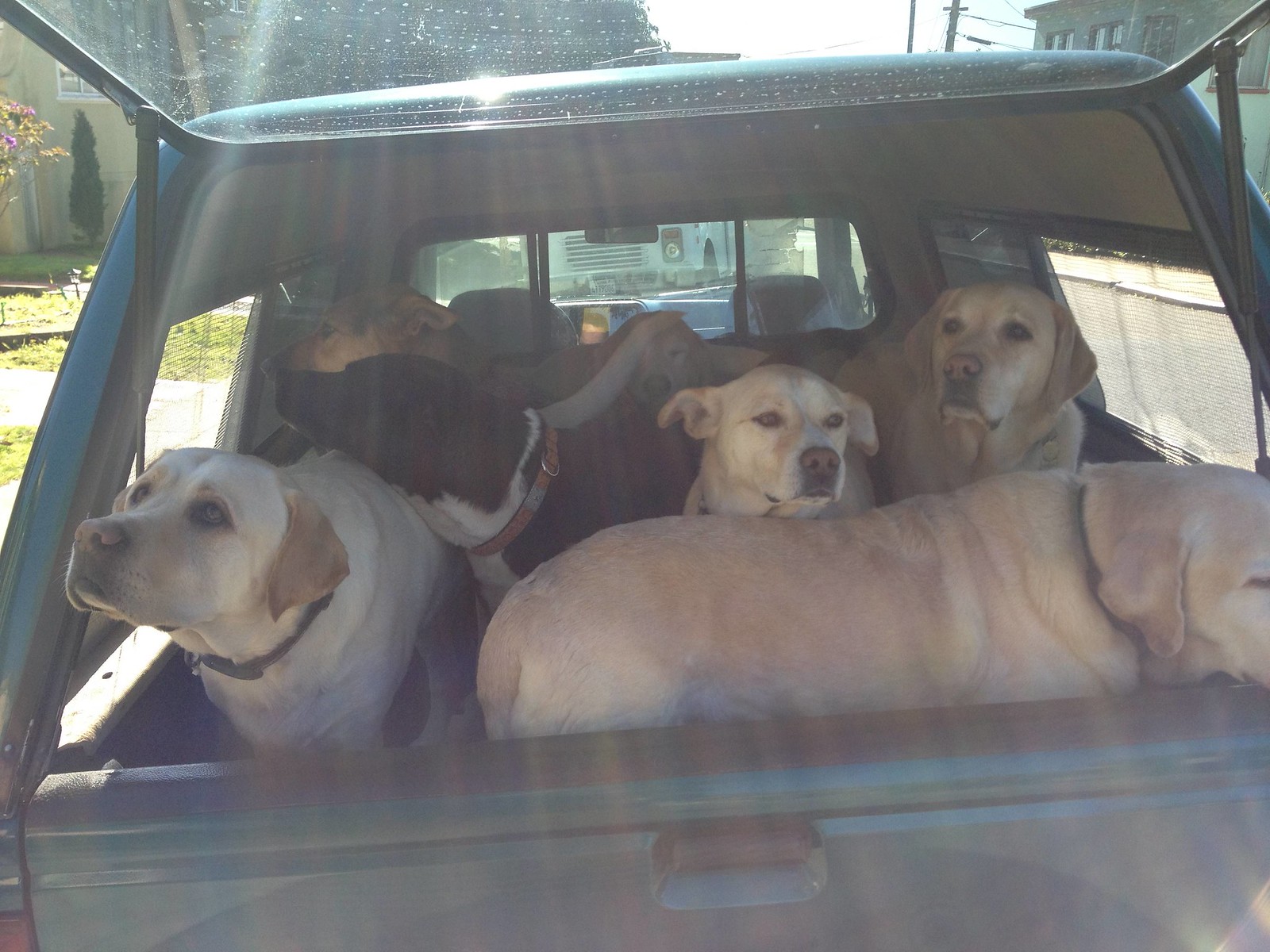This photograph captures a vibrant scene featuring seven Labrador Retrievers grouped together in the back of a black teal truck with its hatchback window open. The setting is outdoors, with buildings, grass, trees, and pavement visible in the background. The retractable gate's bottom half remains shut, while the top glass portion is lifted, providing a clear view of the dogs. 

On the left side of the image, a white Labrador with yellow ears and a gray muzzle gazes upwards. At the front right, another whitish-yellow Labrador stands out, and behind it, two more white Labradors with gray muzzles and pink noses look towards the camera. Also visible to the left is a black Labrador with a white chin and a distinct white strand running down its neck, looking to the left. In the far back, a golden-colored Labrador looks into the camera. The overall brightness, enhanced by the sunlight streaming through the open window, adds a lively texture to the scene, capturing the expressive faces and diverse positions of the dogs.